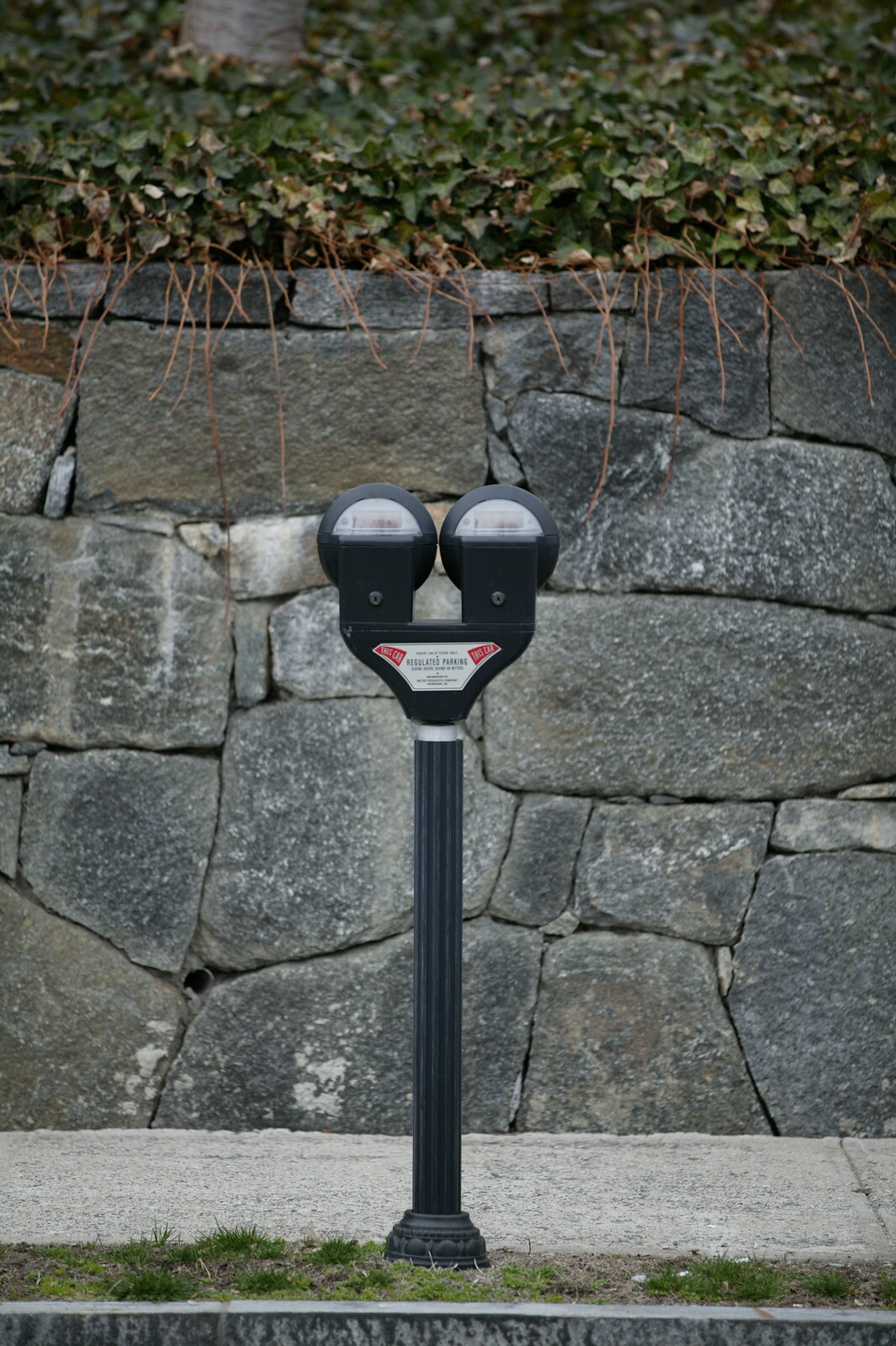In this photograph, a black, dual-side parking meter stands prominently at the center, its base anchored in a small patch of grass. The finely designed base of the meter, resembling a Greek pillar, contrasts with the modern device that rises from it. Two circular meter faces are housed on a flat black top, each adorned with a white and red informational area marked with numbers and instructions. An overcast sky casts a diffused light over the scene, enhancing the details of the background.

Behind the parking meter, a grey sidewalk stretches horizontally across the image, leading to a stone wall. This wall is constructed from irregularly shaped, large stones that fit together in a unique, almost puzzle-like pattern. Ivy climbs along the top of the wall, with green tendrils and brown runners trickling down, seeking new footholds. The combination of natural elements, such as the grass, dirt patches, and ivy, with the man-made structure of the parking meter, presents a quaint urban scene infused with organic textures and patterns.